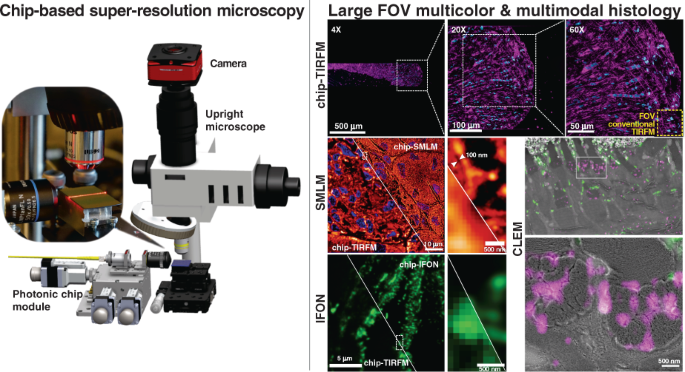The image showcases a sophisticated piece of machinery used for chip-based super-resolution microscopy. The central apparatus includes a camera, an upright microscope, and a photonic chip module, with each part labeled accordingly in black text. The right section of the image features a detailed close-up of the microscope's slide holder, indicating where samples for magnification are placed. Surrounding this central machinery are nine high-resolution close-up images demonstrating the microscope's capabilities, showing various magnified samples with exceptional detail. Additional text highlights terms such as "Large FOV Multicolor and Multi-Model Histology," "IFON," "SMLM," and "chip-TIRFM," which denote different imaging techniques or features of the microscopy system. The machinery and its accompanying descriptions collectively emphasize the advanced nature and high magnification potential of this super-resolution microscopy technology.